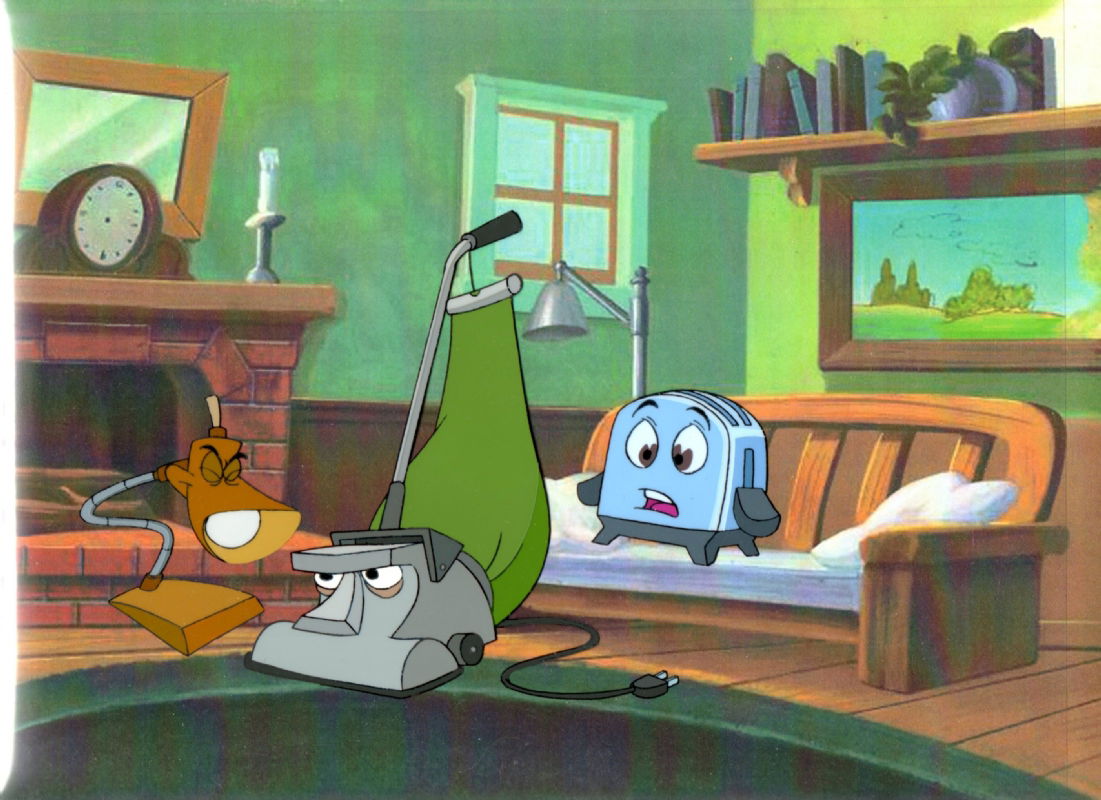This image is a richly detailed still from the animated movie "The Brave Little Toaster," capturing a scene inside a rustic green living room. The walls of the room are painted green, with the lower half adorned in wood paneling. To the far left, a brown-framed mirror hangs above the mantle of a brick fireplace, which holds a wooden clock and a candlestick with a white tapered candle. Logs sit unlit in the fireplace below. On the left side of the scene, a bendable wire lamp with a brown lampshade and a wooden base, animated to appear lifelike, stands with expressive eyes; its light bulb and shade form its mouth and tongue. The lamp seems to be engaging in conversation with an unplugged vacuum cleaner beside it. The vacuum, featuring a green dust bag and a gray handle along with large, emotive eyes, is looking up at the lamp with its back facing a round-top, old-school toaster seated on a wooden couch. The toaster, with a gray base, small legs, and a lever on one side, conveys a look of disbelief or surprise with its partly open mouth. Behind the toaster on the couch, a long blue and green painting in a wooden frame hangs on the wall, while above it, a wooden bookcase filled with books is mounted. The wooden floor is covered by a dark green rug with lighter green edging, completing the cozy, animated scene.